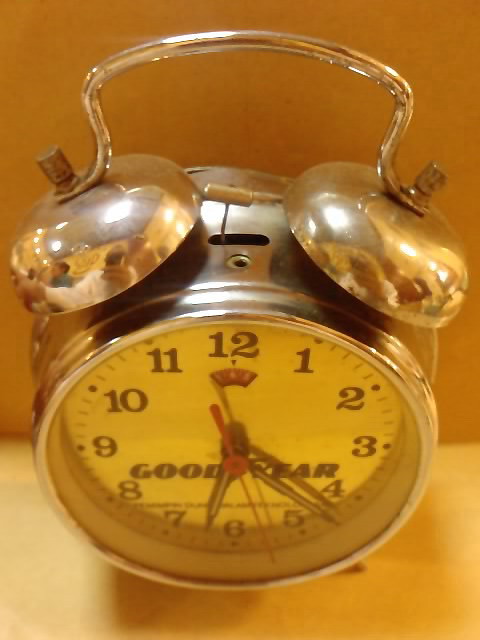This photograph captures a traditional old-fashioned alarm clock set against a dark brown background. The clock rests on a light tan table, viewed from a slightly elevated front angle. The clock itself is circular and made of a silver metallic material, likely steel. Prominently, the clock features two identical round silver bells on the top, each equipped with a knob connected to a metal handle for carrying. Between the bells is a small hammer designed to strike them back and forth to create the alarm sound, reminiscent of scenes from old cartoons.

The front face of the clock is protected by glass and displays black numbers from 1 to 12. Above the number 6, the word "Goodyear" is printed in black, tying in the clock's theme to the Goodyear tire brand. A small red banner is located just beneath the number 12. Completing the clock's design, black minute and hour hands and a red second hand indicate the time on its black and white face. The clock's small feet, though not clearly visible, support its compact stature, making this timepiece a charming nod to classic design.